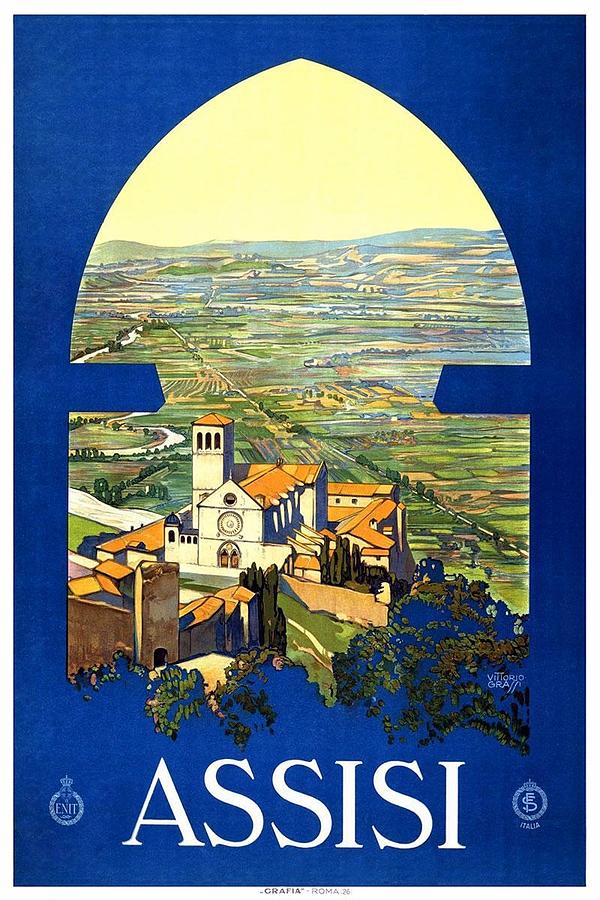The poster features a blue background with an arched window silhouette in the center, showcasing an illustration of the town of Assisi. The illustration depicts a picturesque scene, with a dominant building in the center that resembles a large church, characterized by its white color and orange clay roof. This church-like structure has multiple sections, with one prominent portico rising above the rest. The surroundings include a yellow sky, verdant greens, and detailed roadways, adding depth to the scenic beauty. The base of the poster features the name "Assisi" in large white lettering. Additionally, there are two seals on either side of the illustration, with the right one labeled "Italia." At the bottom center, there is an inscription "Graffia Roma 26" and a signature that reads "Vittorio Gra..." reflecting the artist's name and location.